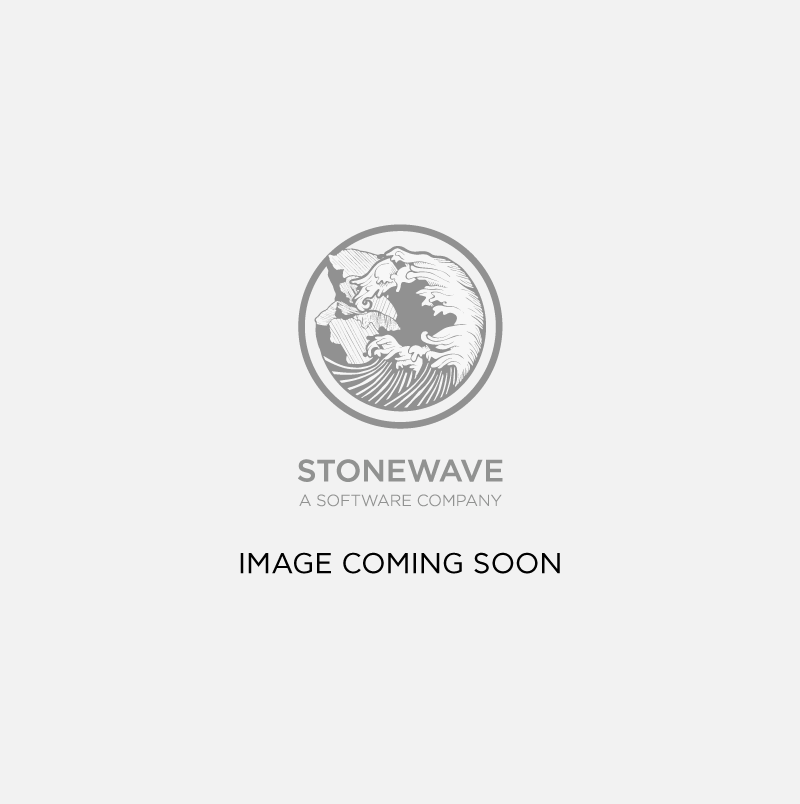This image depicts a piece of jewelry set against a plain white background, featuring a delicate gold chain that loops down from the top. The pendant connected to the chain resembles a blend between a squid and a snowflake, characterized by its intricate, web-like design. The pendant's circular center forms a latticework pattern, creating a semi-transparent effect that contributes to its lightweight appearance. Extending from this center are ten symmetrical, short arms or tentacles, each tipped with small, rounded nubs. The entire piece gleams with a subtle gold shine. Below the pendant, a reflective surface hints at either water or a glossy material, doubling the pendant's intricate design in the reflection at the bottom of the image.